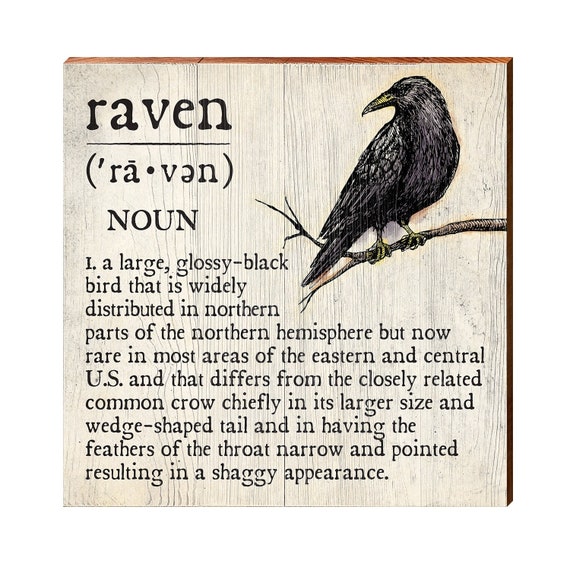This image showcases a detailed engraving on a light, almost whitewashed wooden plaque, possibly repurposed from barn boards. The plaque features a meticulous illustration of a raven perched on a twig in the top right corner. On the top left, the word "raven" is engraved, followed by a pronunciation guide listed beneath it. Below, it states "noun" and provides an extensive definition of the bird. The description reads: "a large glossy black bird that is widely distributed in northern parts of the northern hemisphere, now rare in most areas of the eastern and central US, and distinguished from the closely related common crow chiefly by its larger size, wedge-shaped tail, and the narrow, pointed feathers of the throat giving it a shaggy appearance." This entire detailed depiction, including the bird and the rich definition, is delicately carved into the light-colored wood, giving the plaque an artisanal and rustic charm.